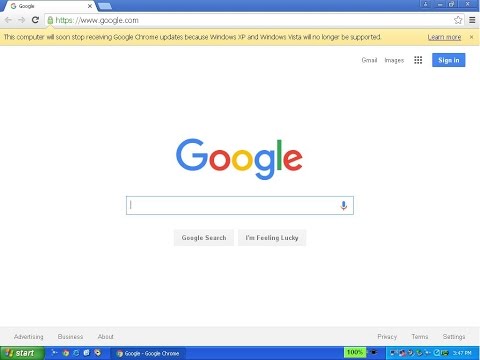The screenshot captures a Google Chrome browser window displaying the Google homepage at Google.com. At the top, the header shows the Chrome browser navigation controls: back, forward, and refresh buttons. The URL bar includes the HTTPS prefix, confirming a secure connection, with the website address Google.com. To the right, there's a star icon for bookmarking. Next to it, under a green padlock symbol indicating a secure site, a yellow notification stretches across the top. It states, "This computer will stop receiving Google Chrome updates because Windows XP and Windows Vista will no longer be supported," alongside a "Learn more" link and a close button (X).

Below this notification, the navigation menu features links to Gmail and Images, a square grid icon for Google Apps, and a blue "Sign in" button. The main section of the page prominently displays the iconic Google logo above the familiar search bar. Within the search bar, options for "Google Search" and "I'm Feeling Lucky" appear, accompanied by a microphone icon on the right.

At the footer, links for Advertising, Business, and About are listed on the left, while Privacy, Terms, and Settings are on the right. Additionally, the Windows taskbar is partially visible at the bottom of the screen, showing the green Microsoft Start button on the left and various application icons, alongside system notifications often referred to as the "Microsoft crap."